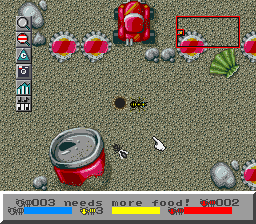A screenshot from a retro-style, two-dimensional video game displays a sandy, beige background, depicting an arid landscape scattered with rocks and a large seashell. Prominently featured is an alert message reading "003 needs more food." The interface showcases a blue bar, a yellow bar, and a red bar, likely representing different character stats such as health, hunger, or energy levels. In the foreground, a distinctive red soda can with an open pull tab stands out against the muted background. Various icons are visible in the corner of the screen, contributing to the game's user interface and hinting at potential inventory items or game mechanics.